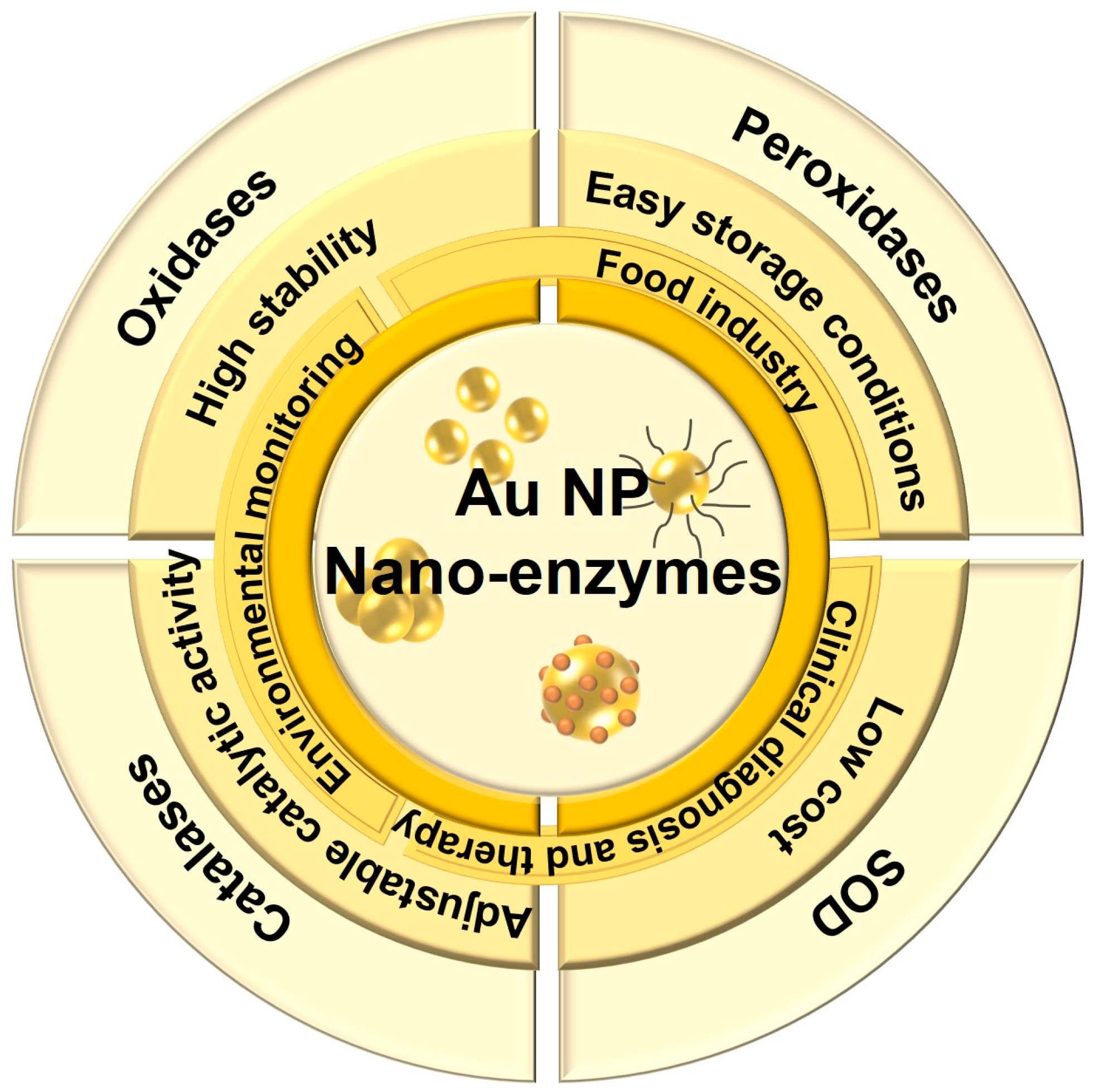The image is a detailed scientific diagram representing the principles and applications of AU-NP nano-enzymes. The central focus is a composition of circles emanating outward in layers of various colors from the center. At the core, in black text, are the capital letters "AU" and "NP" on the first line, and "nano-enzymes" on the second line. The outermost circle is divided into segments, each quarter representing different functions and characteristics of these nano-enzymes. Text labels around the circumference include "oxidases," "peroxidases," "SOD," "catalases," "high stability," "easy storage conditions," "low cost," "adjustable catalytic activity," "environmental monitoring," "food industry," and "clinical diagnosis and therapy." Additionally, the diagram includes graphical illustrations of four types of nano-enzymes: independent golden balls, golden balls joined together, a golden ball with black hair-like projections, and a golden ball with small red balls attached to it. The image uses a palette of off-white, yellow, and orange hues to highlight the different sections and layers, resembling an illustration of a human cell or an earth cross-section.